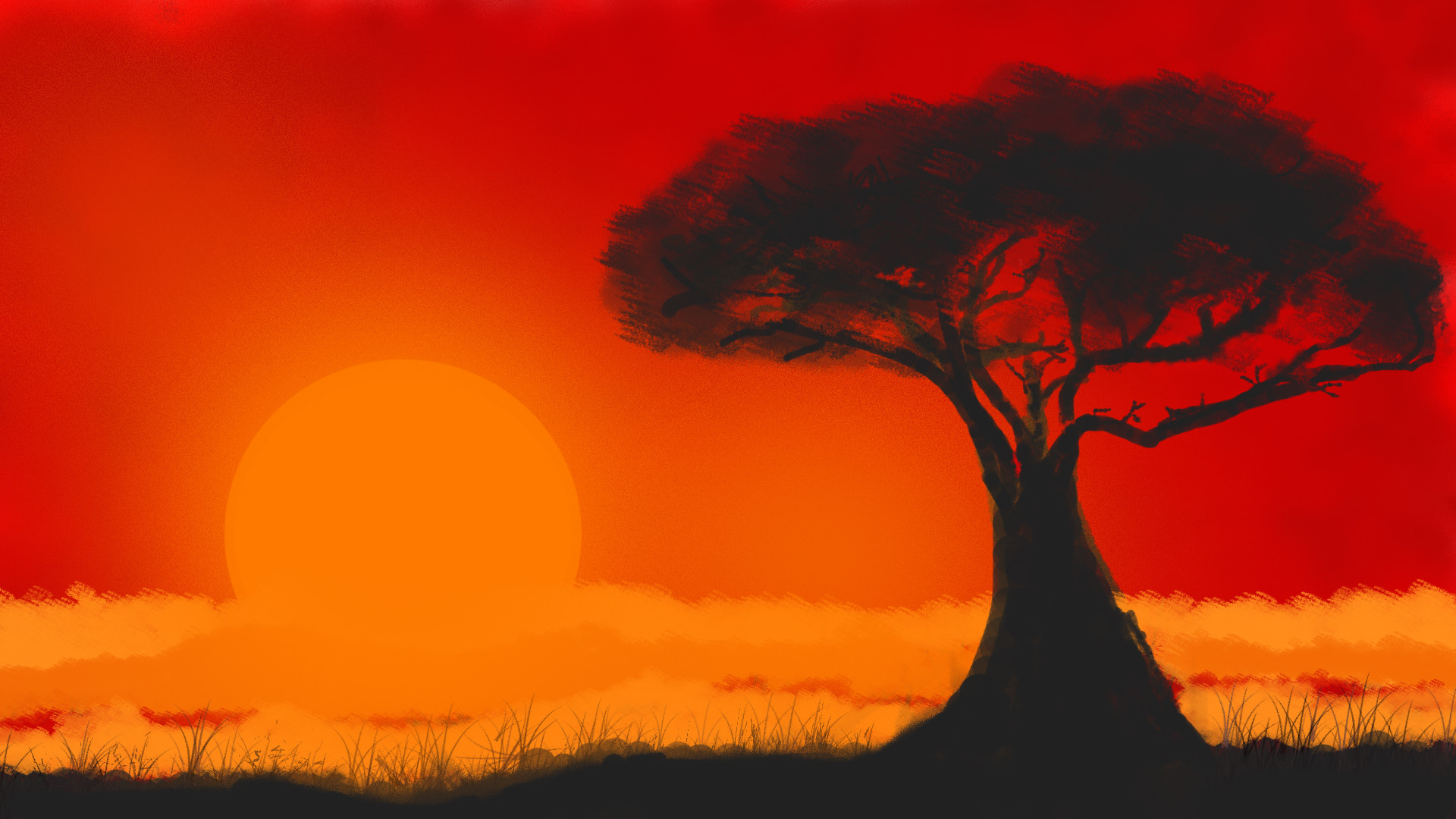This vivid computer-generated image captures a stark contrast between dark and vibrant hues. Dominating the right side is a robust tree trunk that gradually narrows as it ascends. The thick branches extend outwards, adorned with leaves that appear in various shades of black, creating a silhouette effect. The bottom of the image is enveloped in darkness, with slender, shadowy blades of grass reaching upwards.

The upper three-quarters of the background burst with a brilliant reddish-orange gradient, intensifying the fiery atmosphere. On the left side towards the lower portion, a circular glow of light orange adds a focal point of intrigue. Below this, the scene transitions into a vivid blend of yellow, orange, and red patches. This section features irregular stripes of orange floating within the yellow, coupled with delicate red lines that weave through the yellow, blending seamlessly at their edges. The dynamic interplay of colors and the detailed silhouette create a striking visual effect that draws the observer in.